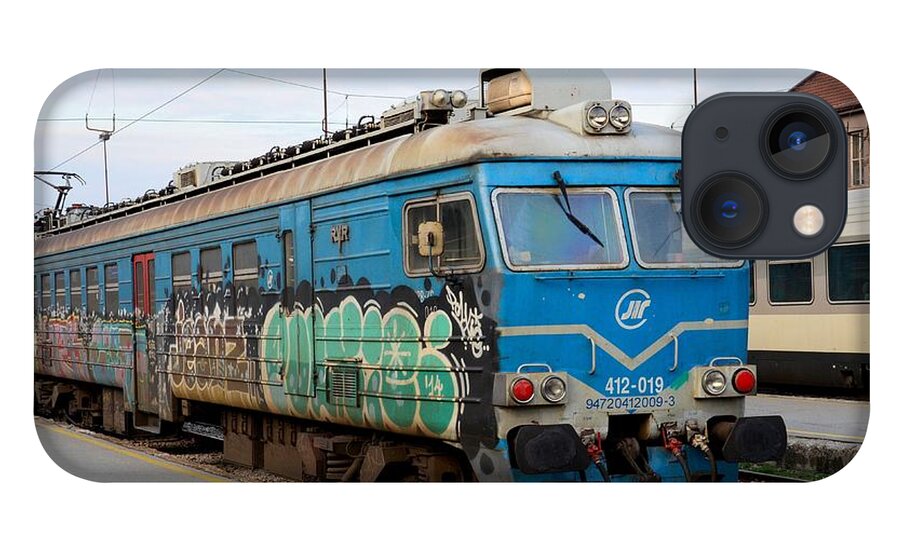The digital image showcases a cell phone case featuring a striking photograph of a vintage train, possibly from the 1960s or 1970s. The phone case itself, with two camera lenses and a flash in the upper right corner, frames the scene against a black background. The train depicted on the case is predominantly blue with a dirty white top, showing signs of age through rust on its wheels and roof. The front of the train, located on the right side of the image, sports the logo "JIR" encircled near its blue and light blue windshield, which has wipers attached. Heavily covered in graffiti, the left side of the train features elaborate tags, starting with aquamarine and white-outlined graffiti transitioning to brown tags with white and black contours, stretching towards the rear. The train appears stationary, with visible electrical lines above indicating it's a trolley. The scene includes surrounding details like a possible station building and various overhead wires, contributing to the authentic, gritty urban atmosphere. The image melds shades of blue, teal, white, black, purple, pink, and green, adding to the vibrant yet weathered aesthetic of the train.